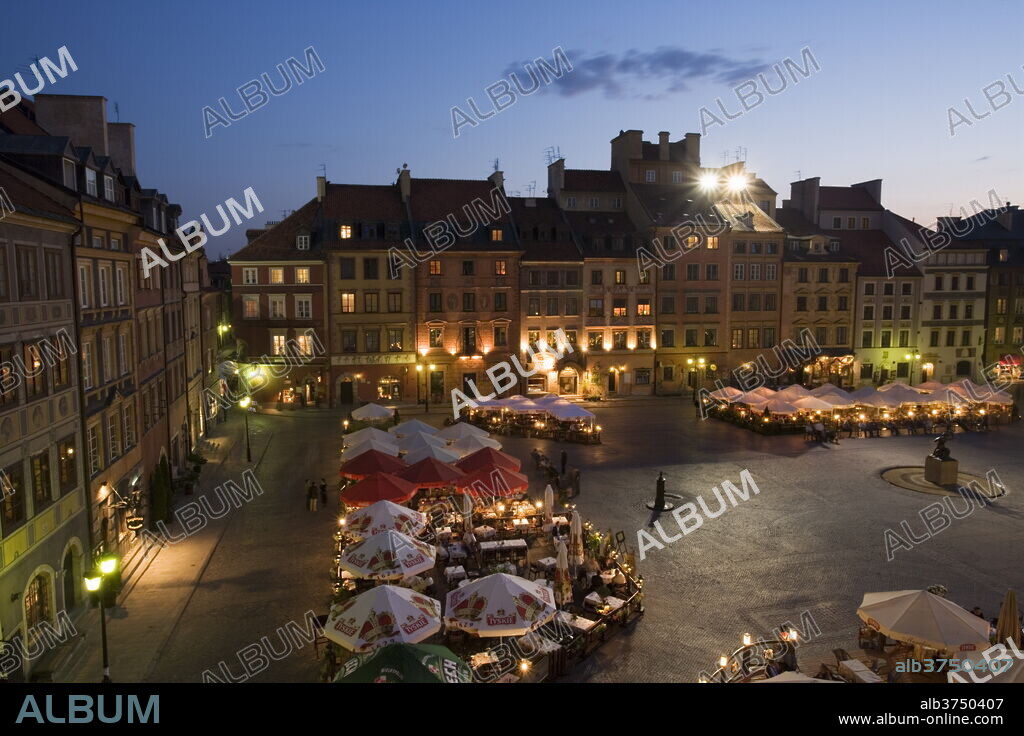This photograph captures a bustling public square surrounded by a cohesive block of tall, four-story buildings made of dark tan brick, creating an enclosed, rectangular space that evokes a distinctly European, possibly German, architectural style. The buildings touch seamlessly with no gaps between them and feature flat facades adorned with rows of windows, lending an orderly aesthetic to the scene. Notably, the structure with a blue hue stands out amongst the otherwise darker spectrum of colors, collectively including another darker blue, a red, and a couple of brownish buildings.

The square is a hive of activity with numerous tables and chairs under both solid red and white umbrellas, the latter adorned with intricate red and gold crown patterns around the edges. Some larger, flatter awnings provide additional shading. People are seen walking and seated, suggesting a lively, communal atmosphere. Light posts sprinkle the perimeter, casting soft illumination as evening approaches.

Adding to the authenticity of the image, there are watermarks repeating the word "Album" alongside a notice at the bottom indicating the website www.album.online.com, asserting ownership of the photograph. A white sculpture sits prominently on a stone base towards the right-middle, adding an artistic element to the otherwise practical setup. The setting sun casts a warm glow over the scene, enhancing its picturesque quality.